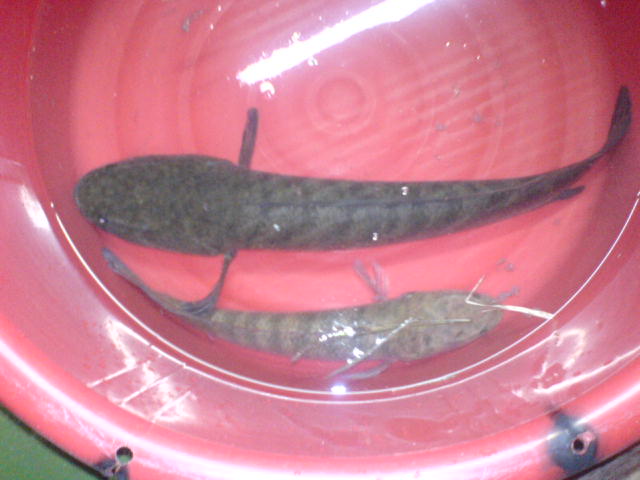The image captures a top-down view of two fish swimming in a water-filled, red-colored bucket. The bucket, about a third full with water, has noticeable holes on its rim with accompanying black marks, suggesting there may have been a rope handle once threaded through. Light shines on the water, making the fish appear shiny as reflections bounce off the surface. The bigger fish, which spans nearly the entire width of the bucket, has a thick head and a smaller tail, with a dark gray to dark green texture. The smaller fish, positioned beneath and facing the opposite direction, is a lighter shade of gray. Both fish resemble catfish. In the lower left corner of the image, a hint of green background can be seen outside the bucket.